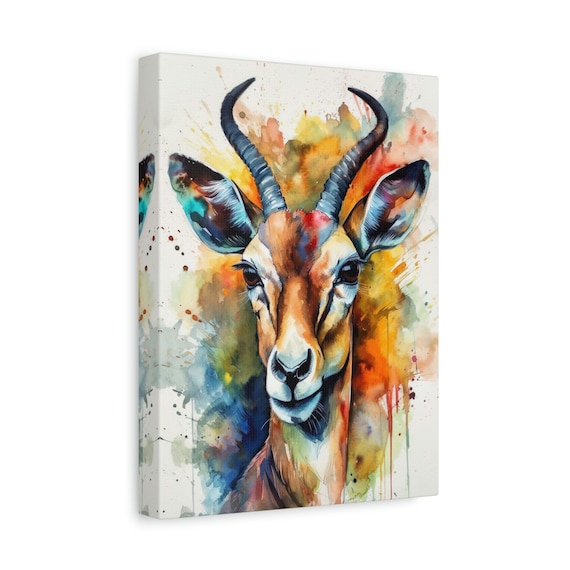The image features a detailed painting on a canvas, mounted on a white wall, depicting a deer with antlers. The deer, facing forward in a portrait style, has a distinctive appearance with brown fur adorned with splotches of various colors including pink, green, and red around its neck. Its face is characterized by a white snout with a black nose and brown eyes, giving it a somewhat blank expression. The deer’s ears, which have white tufts at their base, are colored inside with shades of teal, orange, and black. The background of the painting is an abstract mix of vibrant colors - yellows, blues, greens, and oranges, with the paint applied in a variety of techniques including smudging, layering, splattering, and dripping, adding depth and contrast to the artwork. The entire canvas, even the sides, are painted, giving a vivid and immersive quality to the piece.